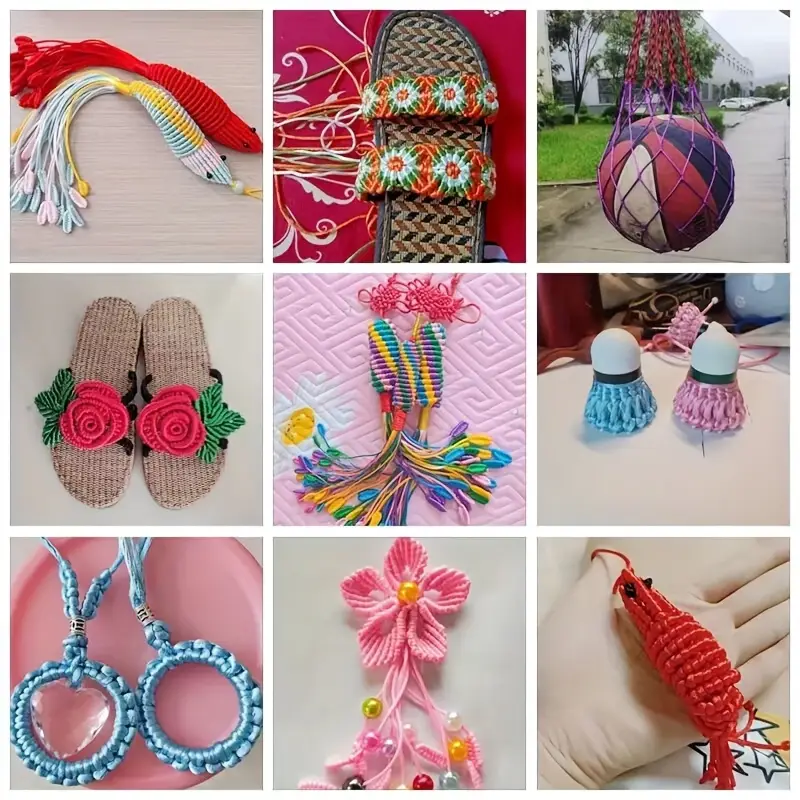This image is a meticulously curated series that features nine square-shaped, equally-sized photographs showcasing various intricate craftworks made from yarn or cord. 

1. **Top Left**: Two yarn-crafted shrimps are depicted. One shrimp is red with a detailed tail and black eyes, and the other is multicolored in white, blue, and yellow.
2. **Top Center**: A macramé sandal with straps decorated by red, green, and orange floral patterns.
3. **Top Right**: A macramé net holding a basketball, hanging in a city street.
4. **Middle Left**: A pair of sandals adorned with woven yarn roses.
5. **Middle Center**: Yellow and purple macramé designed to resemble various party favors or cylindrical whistle pops. 
6. **Middle Right**: Yarn-crafted shuttlecocks, one blue and another purple.
7. **Bottom Left**: Circular earrings made from yarn or macramé.
8. **Bottom Center**: A pink, five-petaled yarn flower with an orange pearl in the center.
9. **Bottom Right**: A red yarn shrimp with black eyes, placed in the palm of a gloved hand.

All images emphasize the versatility of yarn and cord in craft-making, captured in a photographic style across both indoor and outdoor settings.